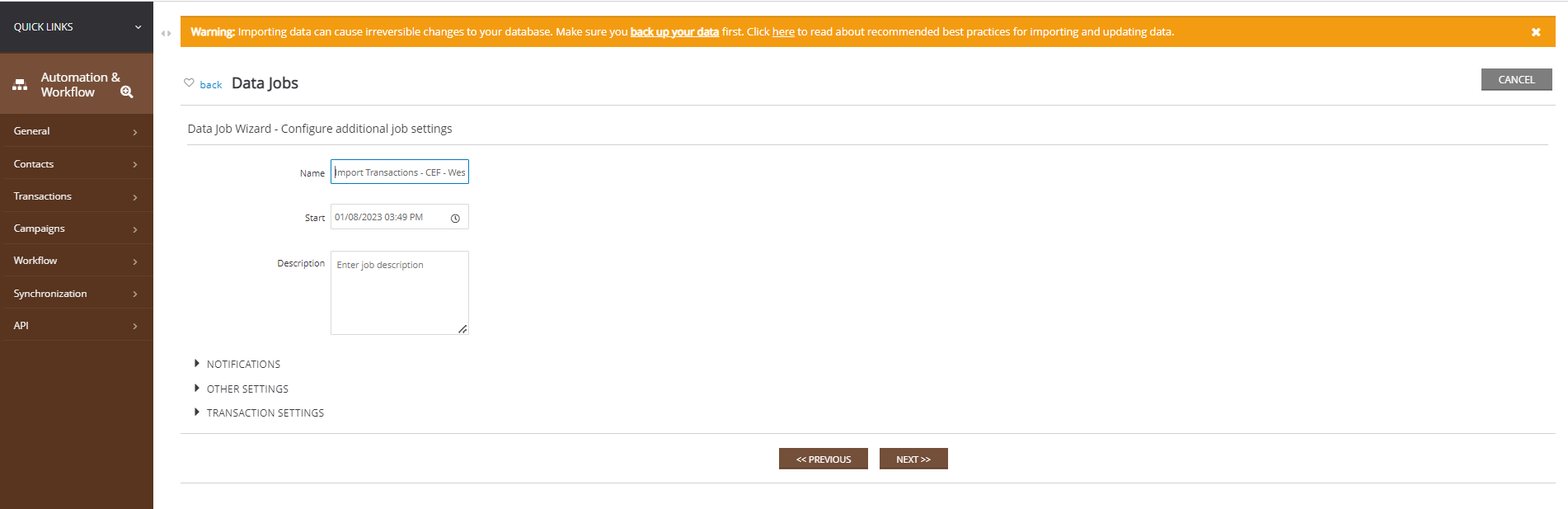**Detailed Image Description:**

The image appears to be a long rectangular screenshot, likely taken from a website. At the top, there is a horizontally extended burnt orange bar containing white text that is somewhat neon in appearance. The only legible word within this text appears to be "Warning," with the rest of the words being too small and indistinct to decipher. On the far right end of this orange bar is a white "X" button.

Below this orange bar, on the left-hand side, is a series of icons and text. Starting from the left, there's a black heart icon followed by a blue icon with indiscernible text. Next to these icons, there are black letters spelling out "Data Jobs." Far to the right, beneath the orange bar and directly under the white "X" button, is a gray button labeled "Cancel" in white text.

Beneath the "Data Jobs" label is another black text reading "Data Job Wizard." Right below that, there's a subtler text line that likely says "Configure Additional Job Settings." Adjacent to this area, there's an input box for text entry, labeled "Name," which currently contains some unreadable text due to its blurry and small size. Further down, there's another label that probably reads "Type," though the text inside the corresponding input box is not clear. The same applies to another box below it that has a small, unreadable text label next to it.

On the lower left side of the image, there are three brownish triangles, forming bullet points, arranged vertically. The top bullet point is labeled "Notifications," the middle one "Other Settings," and the bottom one "Transaction Settings," all in black text.

Towards the bottom center of the image are two brown buttons. The left button, labeled "Previous" with arrows pointing left, and the right one, labeled "Reset" with two arrows pointing right, both in white text.

On the far left side, at the top of the long rectangular section, there's a gray box with "Quick Links" written in white. Below this gray box, the background transitions to a lighter brown, with a section labeled "Automation and Workflow" featuring an unreadable icon to its left. Further down, the brown background gets darker, with a menu header labeled "General." Underneath "General," there are seven clickable boxes with text labels that are too small to read, providing further navigation options. 

Overall, the image is cluttered with very small text, making many elements difficult to fully comprehend.